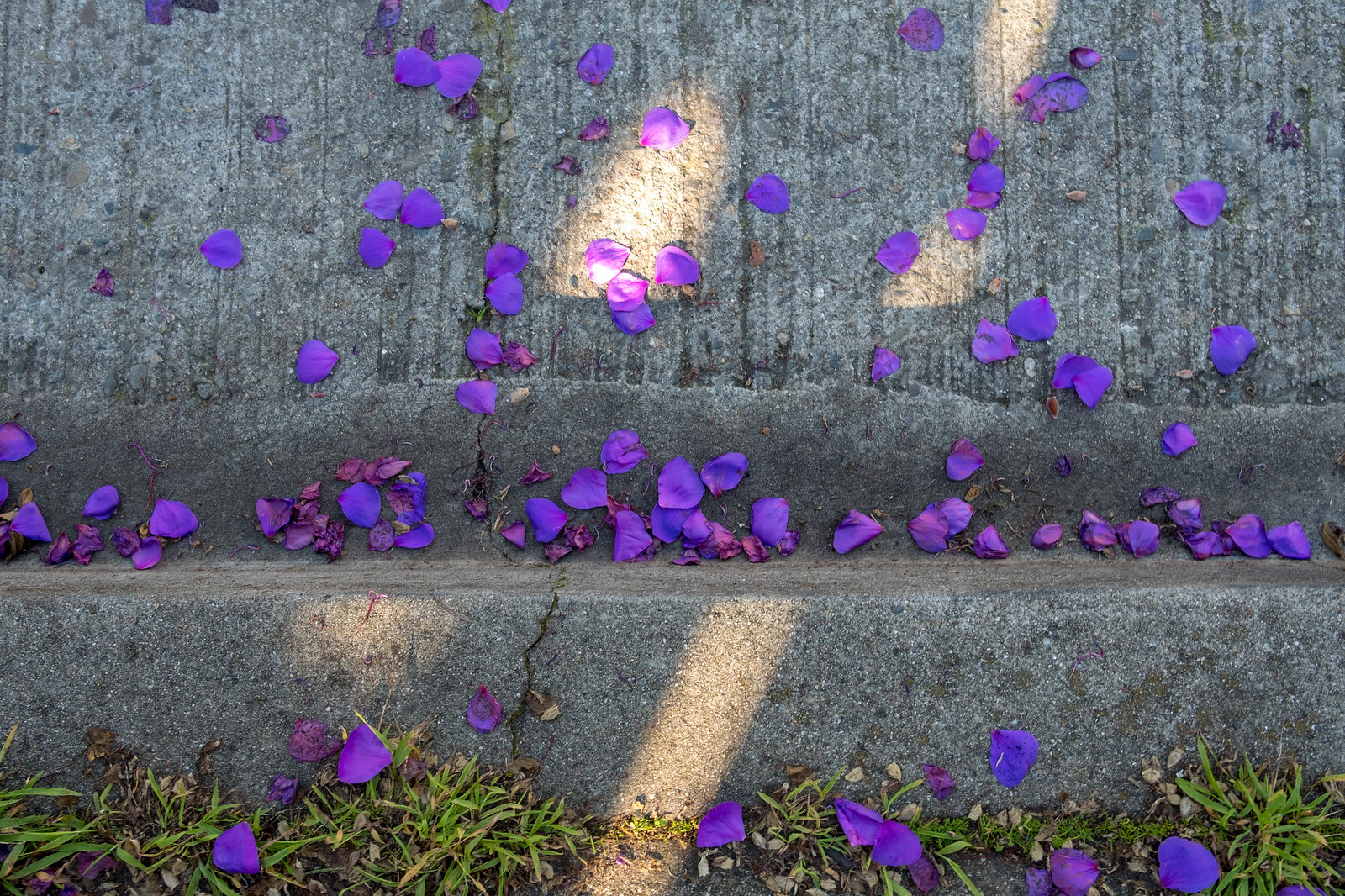The photograph captures an outdoor scene featuring a stone curb and walkway. In the foreground, a patch of grass is visible, followed by a large stone curb that transitions to a slightly elevated stone walkway. Behind this is a short stone wall and a gray wooden fence. Violet flower petals are scattered abundantly across the image—on the grass, along the curb, and covering the stone walkway. The petals are also seen along the edge of the sidewalk and where the walkway meets the next gray ledge. Notably, the walkway and street are marked by distinct cracks; one prominent crack runs along the edge of the sidewalk and intersects with another major crack on the street, forming a Y shape.